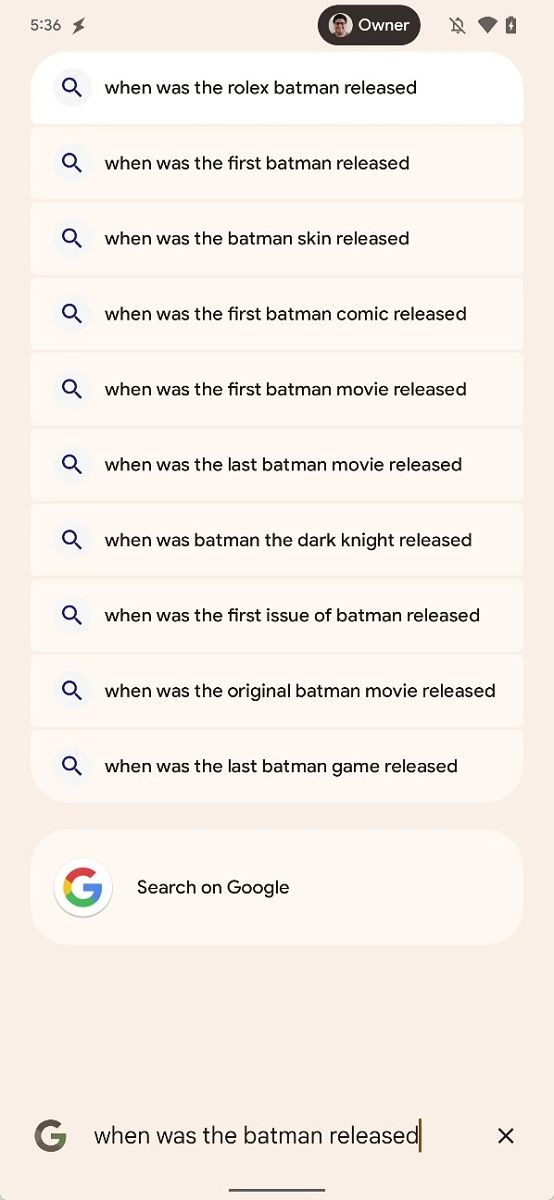A detailed web page displayed on a mobile phone shows various search queries related to Batman. The phone's status bar indicates good battery life, with a lightning bolt icon symbolizing that it's 5:36. An oval profile picture at the top shows an owner with black hair, possibly wearing glasses. 

The main section of the web page is dedicated to a series of questions about Batman, each accompanied by a small image icon on the left. The primary query, highlighted in white, asks, "When was the Rolex Batman released?" Followed by a list of similar Batman-related questions, such as:
- When was the first Batman released?
- When was the Batman skin released?
- When was the first Batman comic released?
- When was the first Batman movie released?
- When was the last Batman movie released?
- When was Batman the Dark Knight released?
- When was the first issue of Batman released?
- When was the original Batman movie released?
- When was the last Batman game released?

Centrally positioned on the webpage is a search box displaying the multicolored Google "G" icon with the prompt "Search on Google." At the bottom of the page, another search query appears, "When was the Batman released?" followed by a gray Google "G" icon. The overall background color of the webpage is a light peach tone.